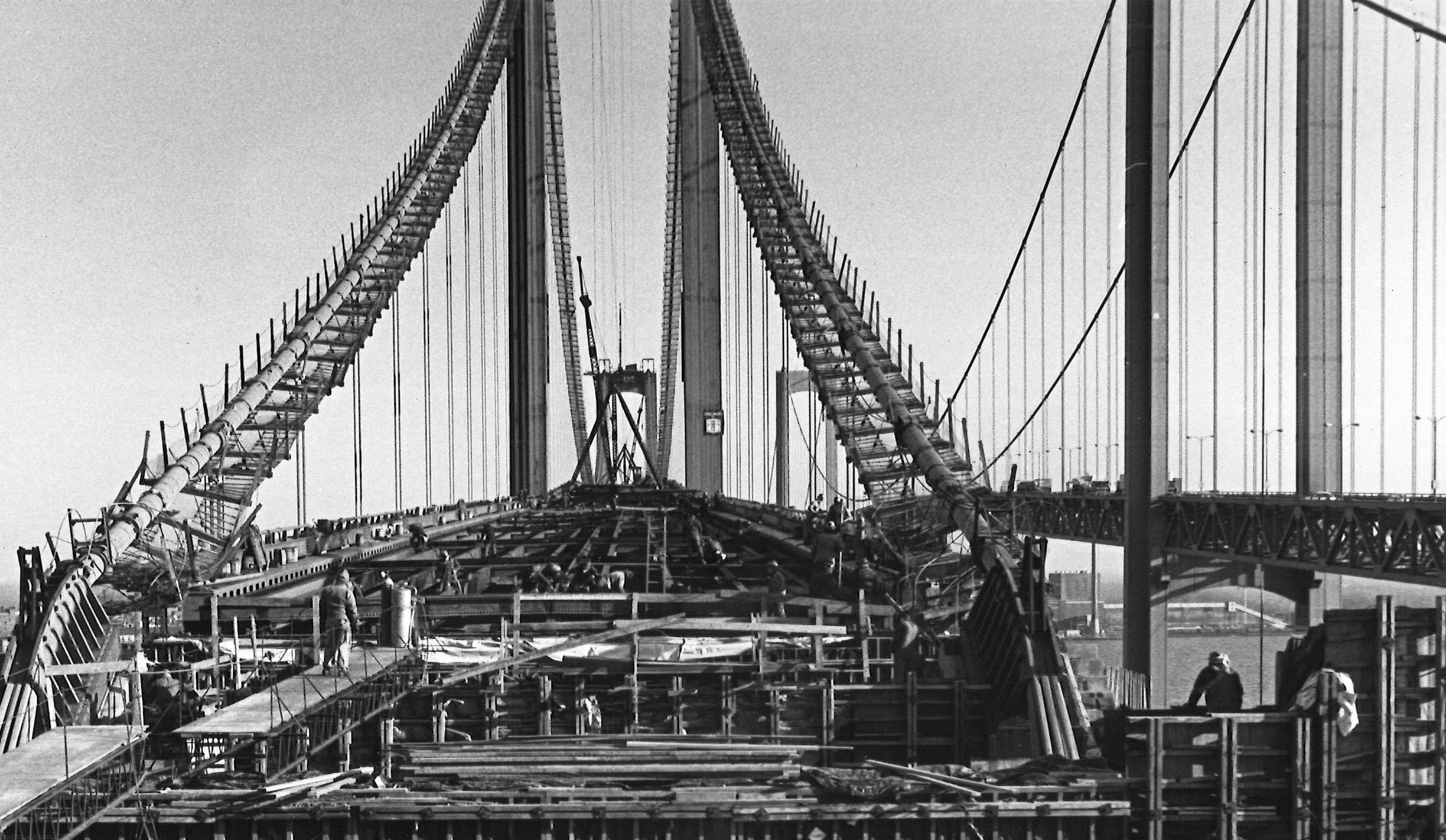This detailed black-and-white photograph captures the intense construction phase of what seems to be a massive suspension bridge, potentially the Golden Gate Bridge based on its riverside location with a cityscape in the background. The photograph focuses on the left side bridge, which is still under heavy construction. The primary suspension cables already rise majestically from the left and right sides of this incomplete structure, while numerous workers are diligently laboring on beams and temporary walkways amidst an intricate criss-cross pattern of steel support columns and planks. These structures run both lengthwise and widthwise, offering a glimpse into the robust framework that will eventually support the roadbed. The bridge on the right appears fully operational, with vehicles traversing it, contrasting sharply with the skeletal form of its twin under construction.